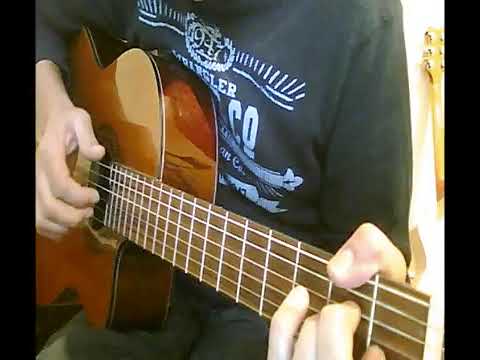The image is a medium to close shot featuring a person actively playing an acoustic guitar. The individual's head is cropped out, leaving only their torso and lap visible. They are seated and wearing either blue or gray jeans, along with a dark gray or black long-sleeve shirt adorned with white text and possibly a Wrangler logo. Their right hand is seen strumming the shiny, reflective brown body of the guitar with fingers, rather than a pick, while their left hand presses down on the fingerboard. A second guitar is noticeable, leaning against a light-colored wall just over their left arm. The background includes a small strip of light hitting the wall behind the player and a slim black border on each side of the picture.